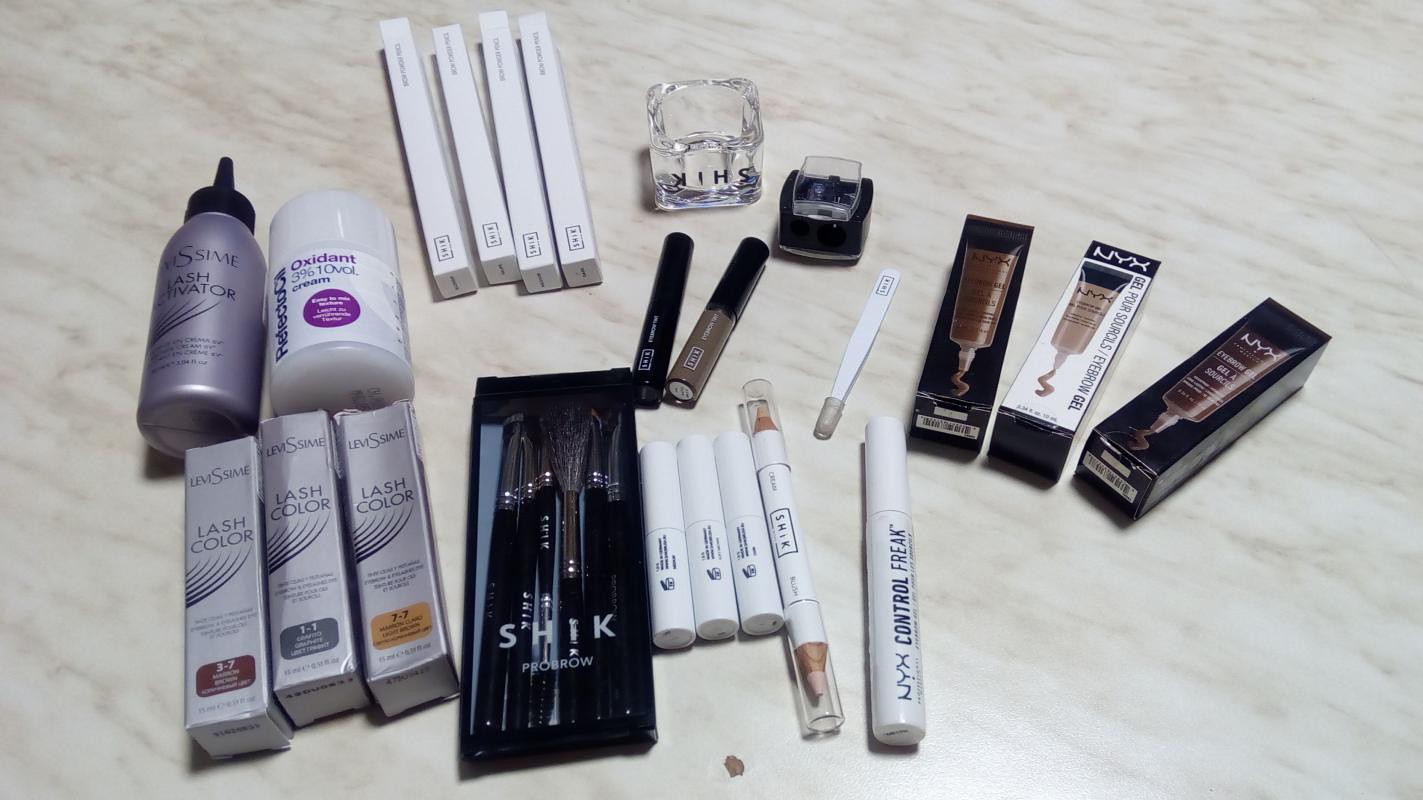The photograph showcases a meticulously arranged collection of beauty products on a glossy white marble-like tabletop, creating an elegant and organized display. On the left side of the image, there are three silver boxes from the brand Levesime, each labeled with a different lash color. The box on the left features a brown logo indicating a brown lash color, the middle box is silver, and the right box has a light brown-yellow hue. Above these boxes lies a purple metallic bottle, possibly plastic, labeled as a lash activator from the same brand, positioned horizontally.

Adjacent to the lash activator is a white tub with a screw lid labeled as oxidants, 3% 10 volume cream from the brand Reflectacil. Moving further right, at the top of the image, there are four long, thin white boxes, the contents of which are not specified. Below these boxes is what appears to be the glass top of a bottle, detached and turned upside down beside its black base.

In front of this setup, there are two mascaras, one black and one brown, accompanied by an eye pencil. At the forefront of the image is a bag labeled Schick Pro Brow, containing brow brushes. Next to the bag are three white lipstick-like containers, followed by a brow coloring pencil. Among these items is a pen-like product called Control Freak in white packaging with a white lid, resembling a felt-tip pen intended for lashes.

Finally, on the far right are three boxes from the brand NYX. Although their contents are unclear, the images on the boxes suggest they contain some form of cream or foundation. These NYX boxes are color-coded with two black and one white box completing the arrangement.